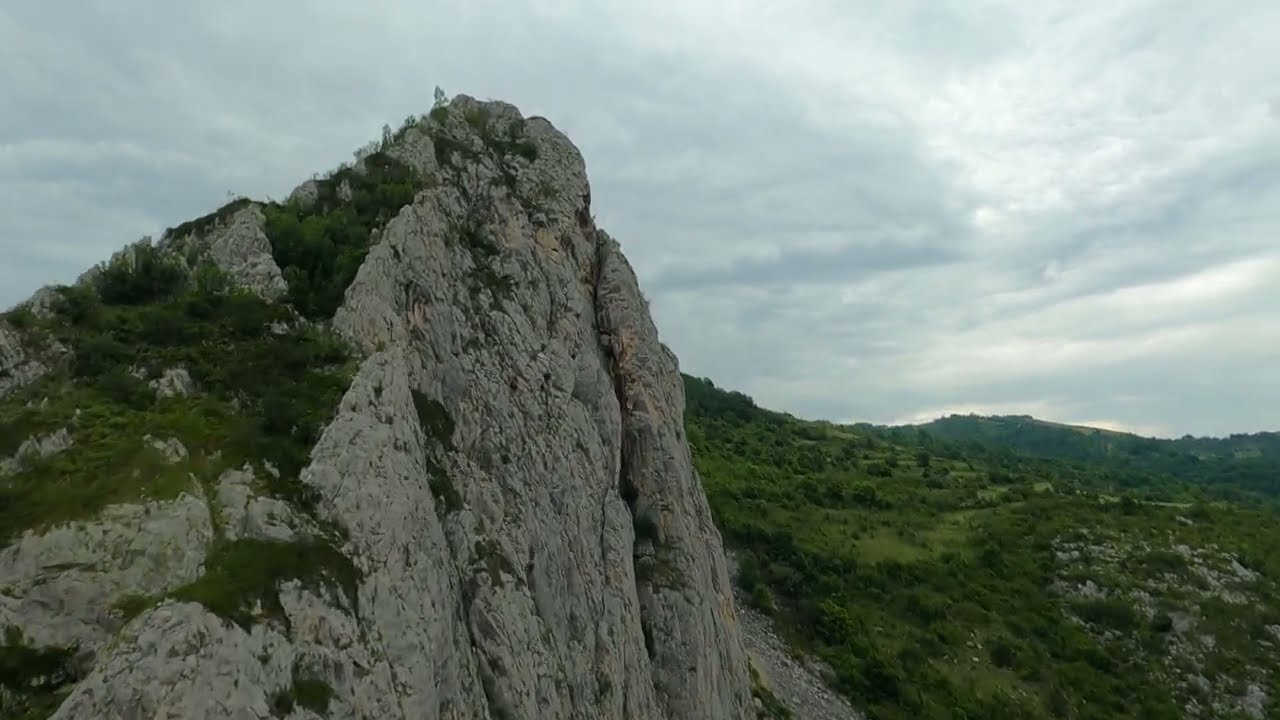A rugged gray rock face dominates the left side of the image, angling steeply toward the light blue sky. Atop this craggy formation, patches of greenery, including grass, moss, and small bushes, cling to the nooks and crannies, enlivening the harsh stone surface. The sky is overcast with streaks of sun piercing through the clouds, casting a gentle light over the scene. Below and to the right, the landscape transitions into a sprawling valley, rich with greenery and broken by areas of gravel and rocky terrain. In the distance, additional mountainous regions rise, covered with shrubs and grass, adding depth and vibrancy to the image. Despite the heavy cloud cover, the scene captures the rugged beauty of the natural landscape with its interplay of rock, foliage, and open sky.